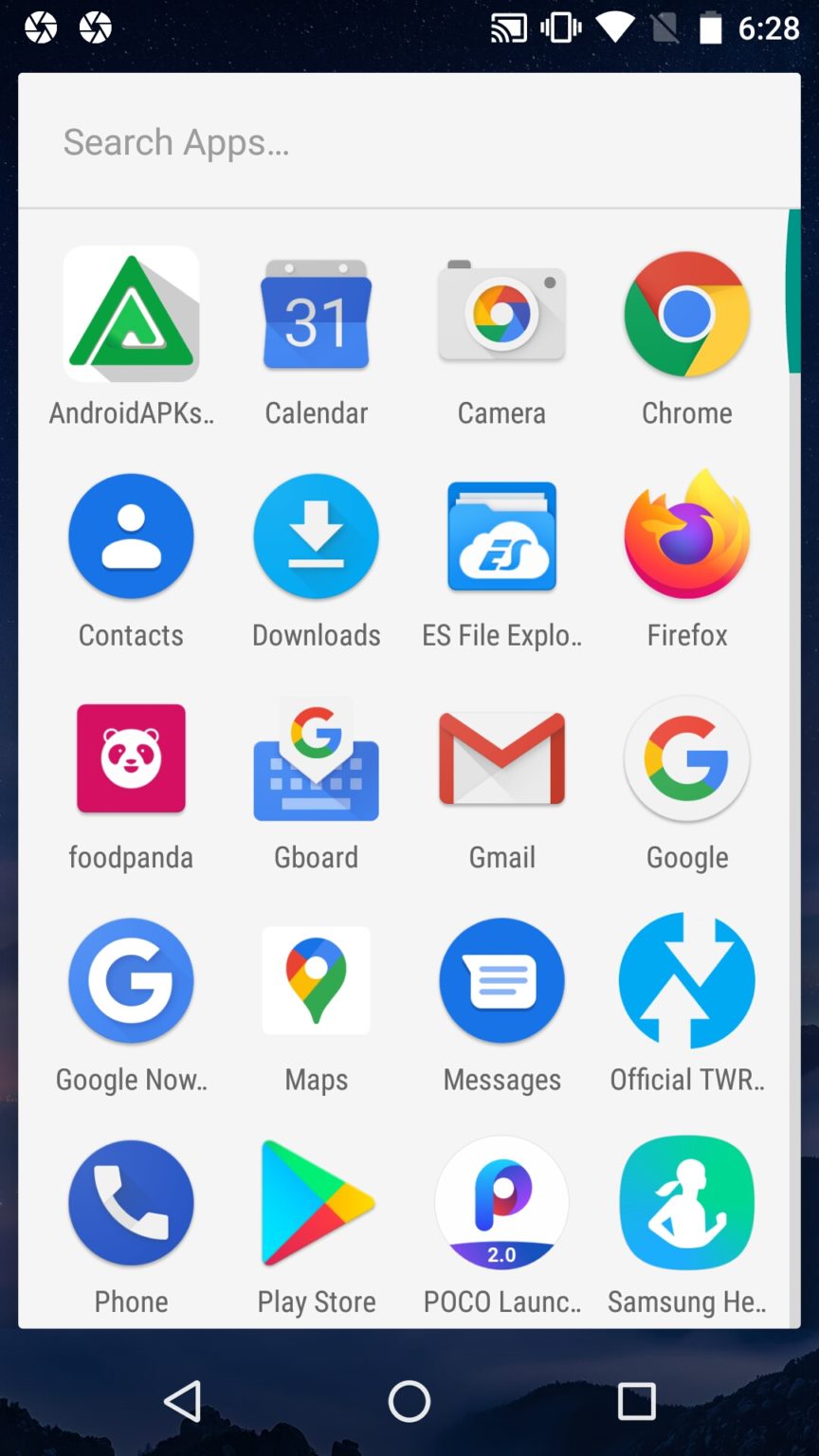The image depicts a screenshot from a cell phone's app page. The phone's status bar, located in the black area at the top, shows the current time in the upper right corner. The borders of the screen are black, framing a vertical rectangular display with a gray background. This central area showcases a grid of 20 app icons.

At the top left corner of the gray background, there is a search bar labeled "Search apps." Below, the app icons are neatly arranged. Some of the easily identifiable apps include:

1. A blue square with a "31" and the label "Calendar"
2. An icon resembling a camera with the label "Camera"
3. The Google Chrome logo labeled "Chrome"
4. The Firefox logo labeled "Firefox"
5. A regular Google logo with the label "Google"
6. An envelope icon with a red 'M' labeled "Gmail"
7. A blue circle with a phone icon labeled "Phone"
8. A red-pink circle with a panda face, labeled "Food Panda"

These icons correspond to various applications installed on the device, providing a snapshot of the phone's home screen layout.